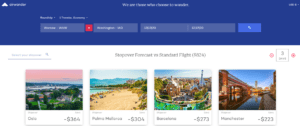The image is a small, blurry screenshot, making discerning details challenging. However, certain elements are still recognizable:

At the very top, there is a dark blue bezel with a white logo resembling a teepee. Adjacent to the logo, there is some white text. In the center of the screenshot, more white text is visible, which appears to describe various sections of what seems to be a travel website, although the clarity is insufficient to confirm this.

Below the central text, there are multiple rectangles, likely designated fields for inputting destinations. The first section includes white text and a recognizable red box with a right-pointing white arrow, suggesting navigation between 'from' and 'to' destinations.

On the right side of the image, there is a mirrored setup with fields likely for searching specific destinations, featuring white text on the left-hand side. Adjacent to these fields, there's a dark blue clickable button with two small, unclear white squares.

On the left, there is a search bar containing gray text and a magnifying glass icon with a gray shadow. 

In the very center, some text is faintly visible, potentially spelling "S-E-O-P-O-V-V-E-F-O-R-R-C-A-S-T" or something resembling "forecast", though the exact text is undiscernible due to the blur.

In the mid-section of the screenshot, there's a gray square with a "3" inside it and two red markings outside of it.

The bottom section contains a series of images depicting various landscapes:

1. The first image features a gradient sky transitioning from pink to dark blue with numerous green trees and is labeled "364."
2. The second image shows a tan and brown beach with blue mountains, dark and tan trees under a foggy overcast sky, labeled "304."
3. The third image displays a cityscape with brown and red brick buildings, some green trees, and overcast blue and white skies, labeled either "273" or "773."
4. The final image illustrates a canal bordered by red and brown buildings under a dark blue sky, labeled "223."

Despite the blurriness, these observations provide a detailed overview of the screenshot's content.